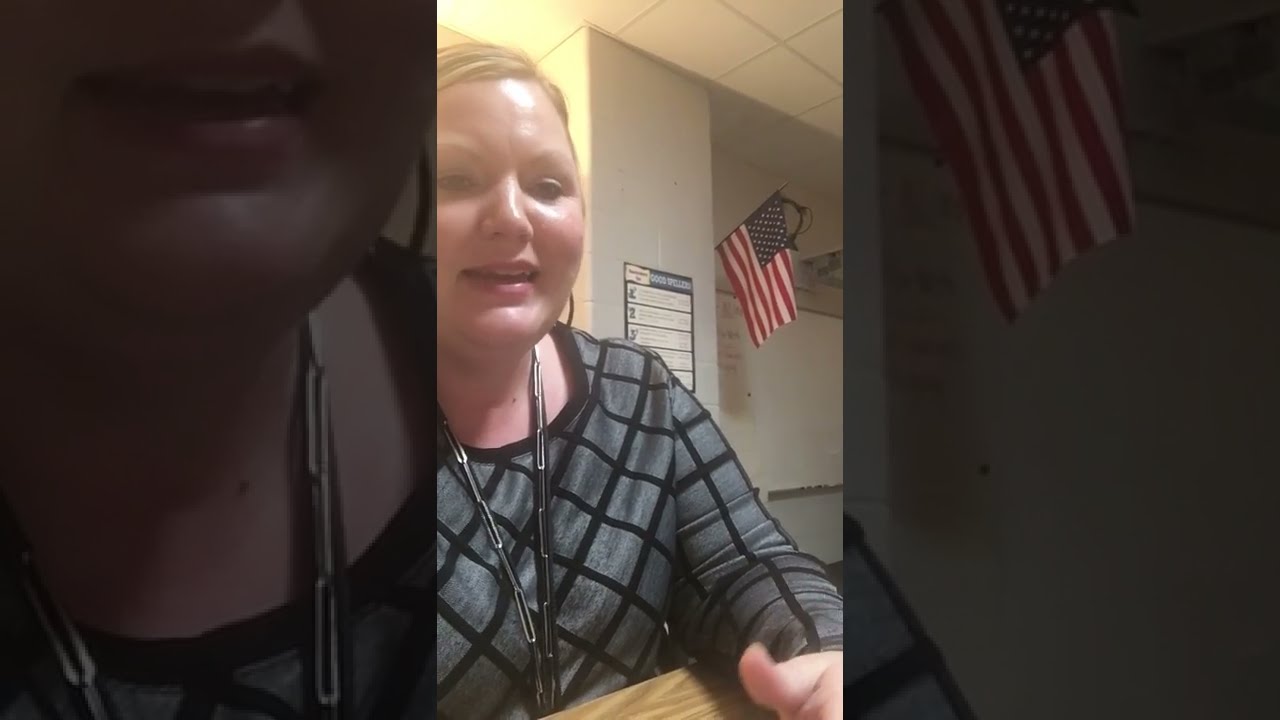A middle-aged woman with fair complexion, blonde hair parted to the side and pulled back, is taking a selfie or possibly recording a video. She has a round face, dark eyes, and pink lips slightly pursed, as if forming a kiss face. She is wearing a black and gray top, possibly a checked t-shirt or sweater, along with a silver, perhaps Bluetooth, necklace around her neck. She is seated in a well-lit room with a white, cinderblock wall in the background. On the wall, there is a black and white poster with writing that is hard to make out, and a bright light source in the upper left corner causing a glare on her forehead. The very bottom right of the image shows the back of a chair.